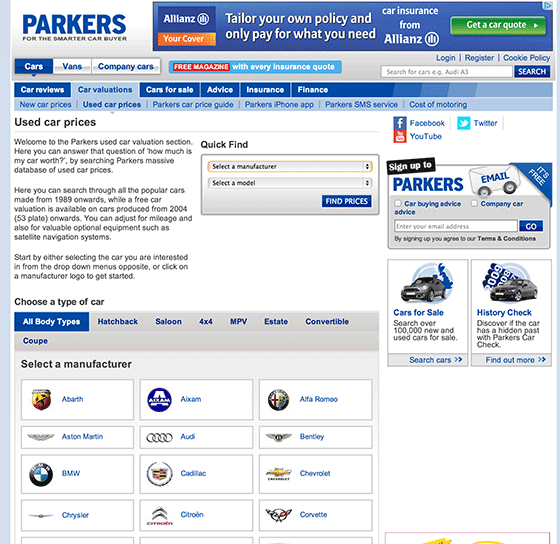**Descriptive Caption:**

The image shows a car buying webpage interface designed to help smarter car buyers. The top left corner of the page features the site's name in blue text. The top right corner prominently displays the Allianz logo, with the slogan "Your Cover" written in orange. The rest of the text is white against a blue background, emphasizing the tagline: "Tailor your own policy and only pay for what you need. Car insurance from Allianz."

A blue button labeled "Get a Car Cost" is situated prominently on the page. On the left side, a sidebar menu includes options such as Cars, Vans, Company Cars, with "Cars" selected. Additional links provided include Cars Reviews, Car Evaluation, Cars for Sale, Advice, Insurance, Finance, New Car Prices, Used Car Prices, Packers, Car Price Guard, Packers iPhone App, Packers SMS Service, and Cost of Motoring. 

The section for used car prices welcomes users to the Packers Used Car Valuation section. It offers the capability to answer the query "How much is my car worth?" by searching through a comprehensive database of used car prices. The database includes popular car models from 1989 onwards and provides free car valuations for models from 2004 onwards. This section allows users to adjust for mileage and optional equipment such as satellite navigation systems. Users can start their search by selecting a car from drop-down menus or by clicking on a manufacturer logo.

On the right side, there is a "Quick Find" option with blue buttons for selecting a manufacturer and a model. Below, there is an opportunity to sign up to Packers with an email.

At the bottom of the page, various car brands are listed under "Cars for Sale" and "History Check," featuring categories for all body parts and brands including Audi, Aston Martin, BMW, Chrysler, Citroen, Cadillac, Bentley, Chevrolet, Corvette, Alfa Romeo, and more.